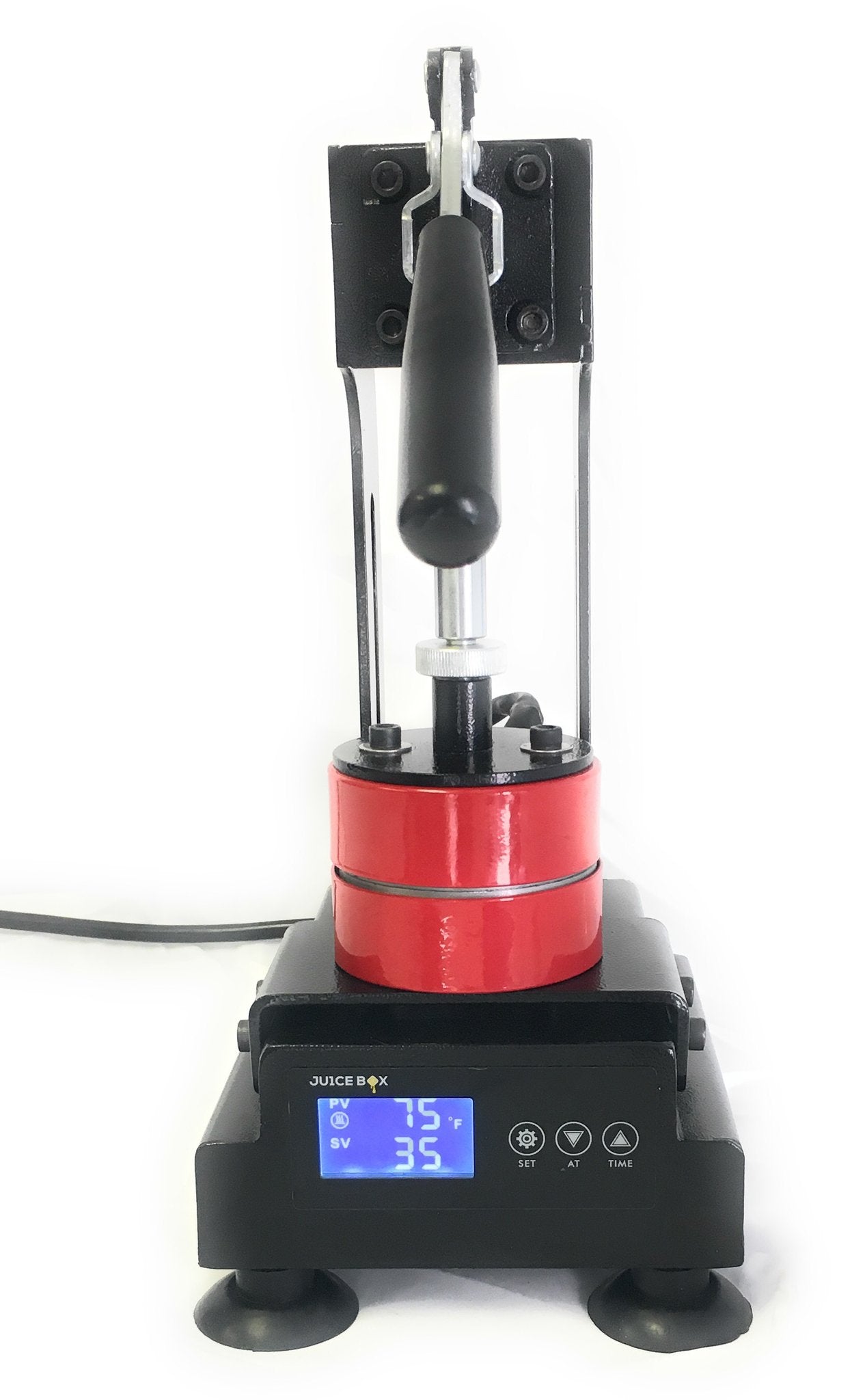The photograph showcases an electronic appliance, explicitly labeled "juice box," against a stark white background. The base of the machine is a sturdy black plastic stand equipped with two black suction cups located at the bottom left and right corners for stability. Prominently displayed on the base is a blue LED screen, which shows the readings "PV, SV, 75 degrees Fahrenheit" and "35." Positioned to the right of this display are three white circular buttons, each with distinctive icons: a gear labeled "set," a downward-facing triangle labeled "at," and an upward-facing triangle labeled "time."

Moving up from the base, a red cylinder is visible, which appears to be part of the pressing mechanism of the juicer. Above this cylinder, there is a glass case encasing a metal tube, adding a transparent segment to the appliance. Topping the machine is a black rectangular piece secured with four screws arranged in a square pattern, and a black handle protrudes from this top section, likely used to operate the press. The machine is in the closed position and shows no signs of use, such as juice or fruit remnants. The black handle suggests functionality in raising and lowering the press. Overall, the device exemplifies a compact, yet detailed design suitable for juicing operations.